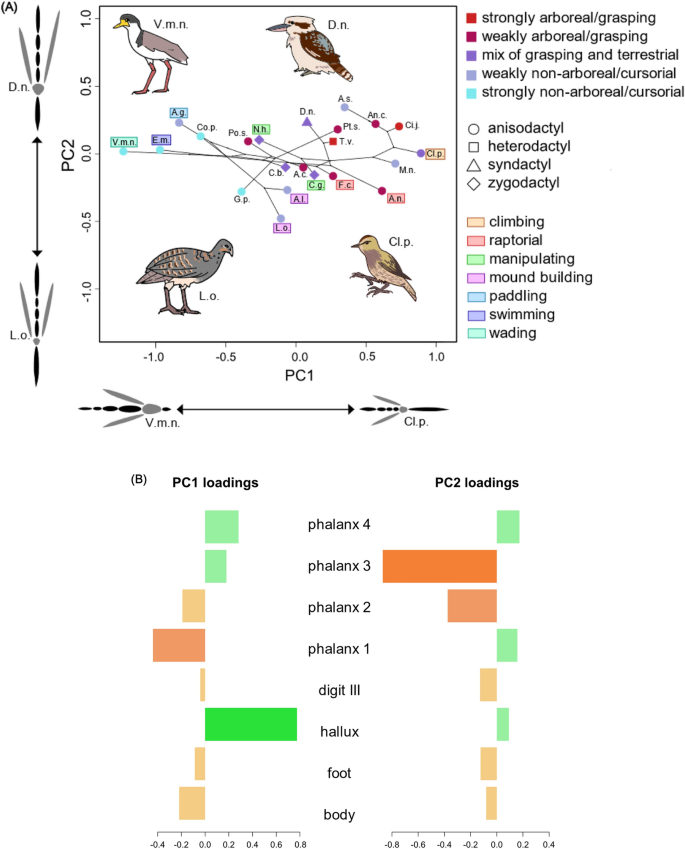The image is an educational poster against a white background, primarily depicting four birds with corresponding labels identifying their species. The top section features illustrations of the birds, each with text to the right specifying their type. Below these images is a colored bar chart in shades of orange, green, and tan, explaining the different activities the birds engage in. Specifically, green signifies waiting, purple indicates swimming, and blue represents paddling. The poster includes various colors—black, white, gray, brown, yellow, purple, pink, green, and orange—correlating to different parts of the chart or illustrations. There are no other objects in the image, emphasizing its educational purpose.